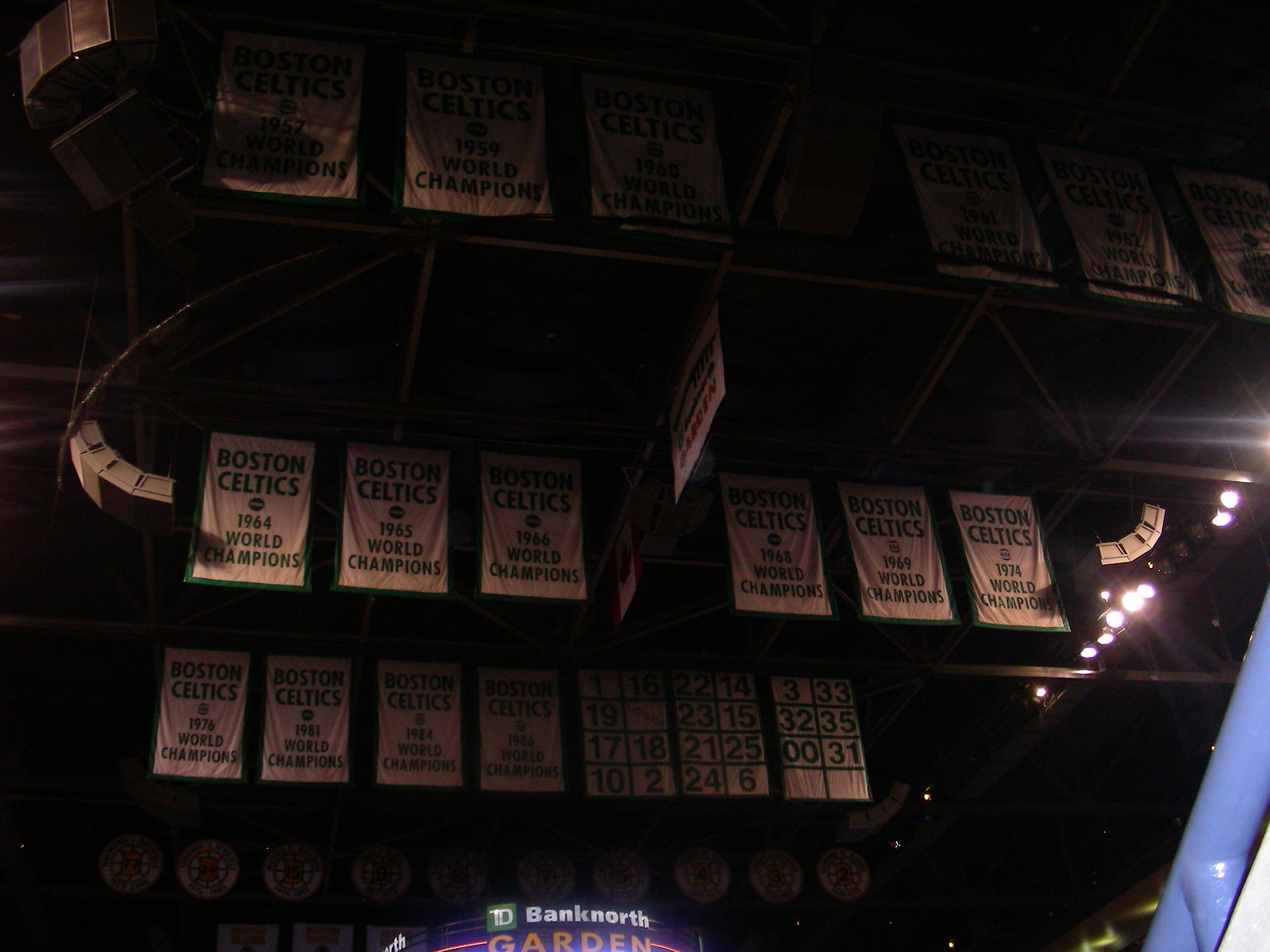This is a detailed picture of the ceiling of an indoor stadium, specifically the Boston Celtics' home arena, known as the Bank North Garden. Dominating the image are rows of green banners celebrating the Boston Celtics' achievements, each prominently displaying titles like "1964 World Champions," "1965 World Champions," and "1976 World Champions." There are three rows of these championship banners, each containing approximately six banners. Alongside these, some banners feature eight sections with two-digit numbers, presumably representing retired jersey numbers or significant years. Positioned centrally and toward the middle right of the image is a cluster of stadium lights, and at the bottom right-hand side is an LED sign on a blue background that reads "Bank North" in white letters and "Garden" in yellow. The bottom part of the image also includes a faintly illuminated blue walkway or an upper section of the stadium, adding to the overall atmosphere of the arena.